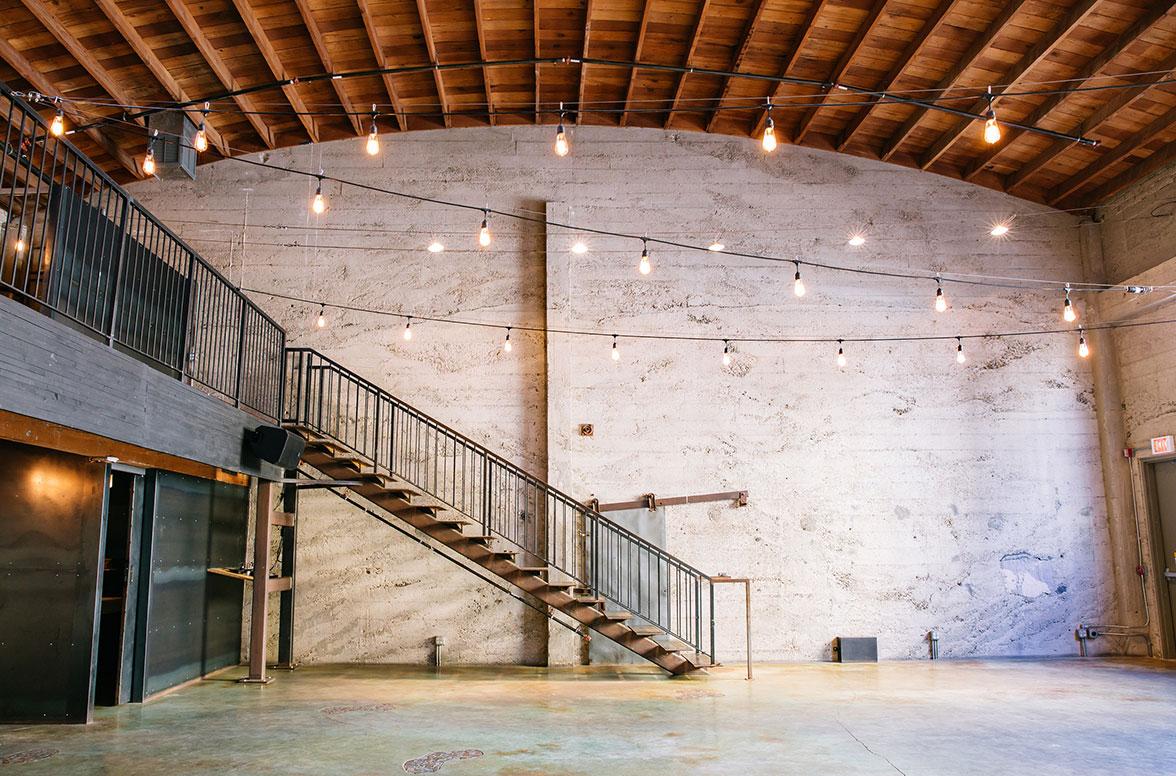The photograph captures a large, rectangular warehouse-like building with a curved ceiling supported by visible wooden rafters. The ceiling appears unfinished, presenting a wooden framework. Below, the floor is a smooth, tan ceramic surface. Inside the space, there is a stairway, equipped with railings, leading to a second level, which features glass-enclosed offices. This second level also has railings around its perimeter. Strings of hanging lights crisscross the ceiling, illuminating the expansive room. On the ground level, there's a black door on the left and an exit door on the far right marked with an exit sign. The building's interior appears bare, with some uncovered concrete walls, contributing to its industrial appearance.